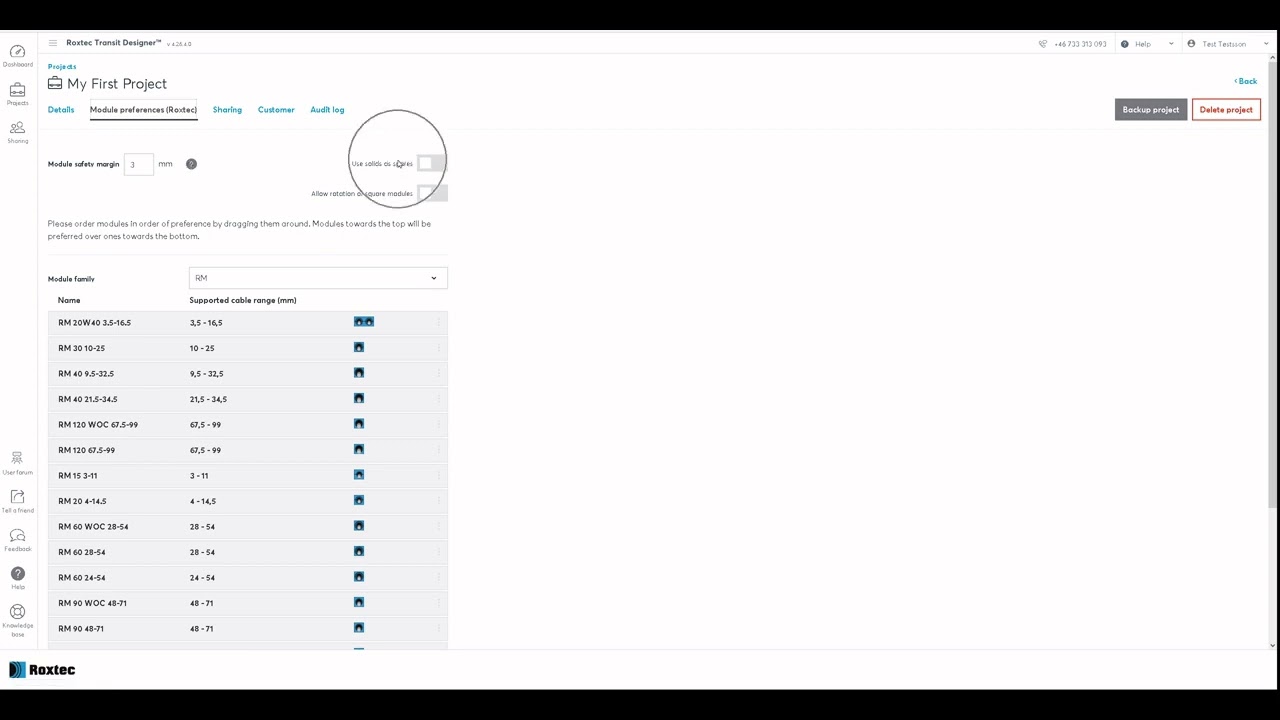This is a detailed screenshot of the Roxtec Transit Designer software interface, specifically from the "Projects" section under "My First Project." At the top of the screen, various tabs are labeled: "Details," "Module Preferences," "Roxtec Sharing," "Customer," "Audit Log," and "Module Safety Margin" with a margin of "3MM."

A prominent area on the screen is circled, highlighting the settings "Use solids as squares" and "Allow rotation of square modules." The instruction is to order the modules in the order of preference by dragging them around, stating that modules positioned towards the top will be preferred over those positioned at the bottom.

Under the "Module Family" dropdown menu, set to "R-M", there are columns designated for "Name" and "Supported Cable Range (MM)." The modules are listed as follows:

1. R-M 20-W 4-0, 3.5-16.5
2. R-M 30, 10-25
3. R-M 40, 9.5-32.5
4. R-M 40 21.5-34.5
5. R-M 120 W-O-C, 67.5-99
6. R-M 120, 67.5-99
7. R-M 15, 3-11
8. R-M 20, 4-14.5
9. R-M 60 W-O-C, 28-54
10. R-M 60 28-54
11. R-M 90 W-O-C, 48-71
12. R-M 90, 48-71

The bottom of the screen features the "ROXTEC" logo in black letters, along with a black bar spanning the width of the image.